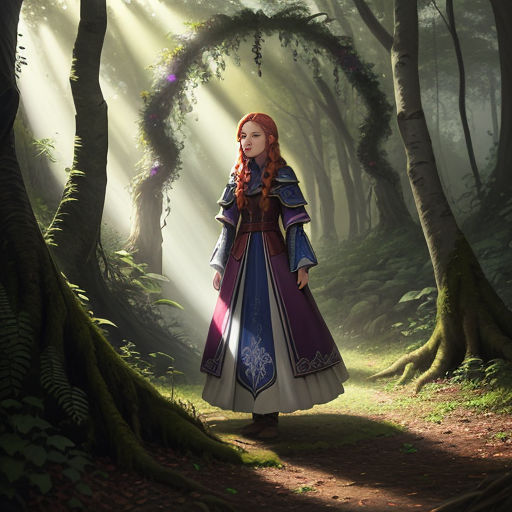This digital illustration depicts a young woman standing on a mossy green path in a dark forest, illuminated by sunlight streaming through the trees from the upper left side of the image. The sun creates a luminous pool of light where she stands, casting her shadow on the ground. Her elaborate dress features multiple layers: a white underdress, an overdress in blue and deep red tones, and intricate shoulder embellishments. The costume includes two sets of sleeves, puffy and dark blue at the top, tapering into frilly wrists. The dress's bottom part showcases a possible crest or floral motif, with hues of blue, red, yellow, and gray. She has striking bright red hair styled in two braids that drape over her shoulders, paired with her pale skin and a somewhat neutral expression. The background is enriched with tall, vine-covered trees forming an arch over the path and accented by purple flowers, while a significant tree stands prominently on either side. The forest canopy creates a dramatic interplay between light and shadow, enhancing the serene yet mystical atmosphere of the scene.